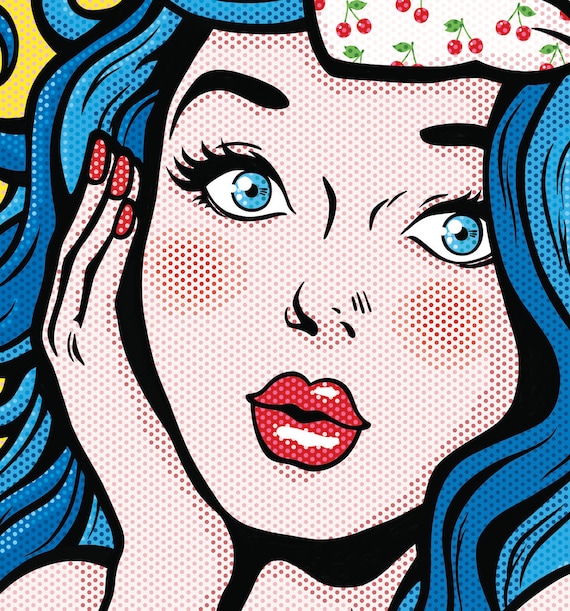The close-up illustration evokes the style of classic pop art comics, characterized by a composition of colored dots reminiscent of vintage printing techniques. It features a striking young woman with ocean-blue hair adorned with a hat decorated with white and red cherries, complete with green stems. Her large, bright blue eyes and big dark black eyebrows draw you into her gaze as she looks directly at you. Her face is framed by pinkish cheeks and pouty, ruby-red lips, with a slight shine enhancing their fullness. She holds her right cheek with her right hand, showcasing her red-painted fingernails, adding to the vibrant palette. The background includes hints of yellow, complementing the primary colors and further grounding the image in a graphic novel or comic book setting.